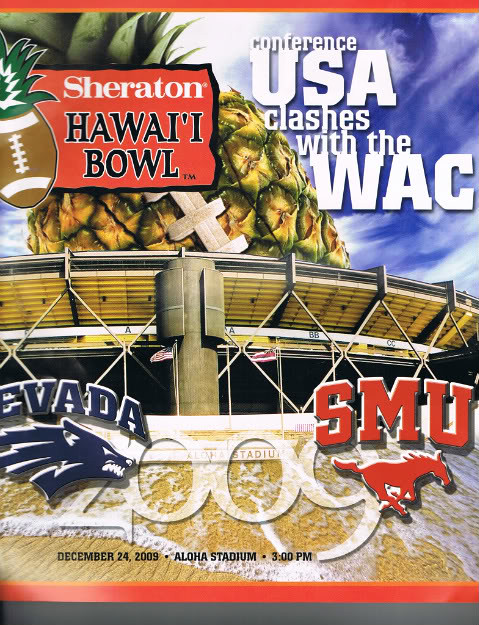This image is a detailed event poster for the Sheraton Hawaii Bowl. Central to the design is a massive pineapple styled like a football, complete with laces and pineapple leaves. Dominating the top of the poster is the title "Sheraton Hawaii Bowl" in white and black print, set against an orange rectangle. Just below this, the text "Conference USA clashes with the WAC" indicates the competing teams. At the bottom, the poster features the logos of Nevada and SMU; Nevada's logo depicts a blue wolf head while SMU's logo showcases a red horse. The date and location details are displayed prominently: December 24, 2009, at Aloha Stadium, 3 p.m. In the background, a blue sky with scattered, swirly white clouds and the seats of a stadium are visible, alongside a beach with waves crashing onto the sand.